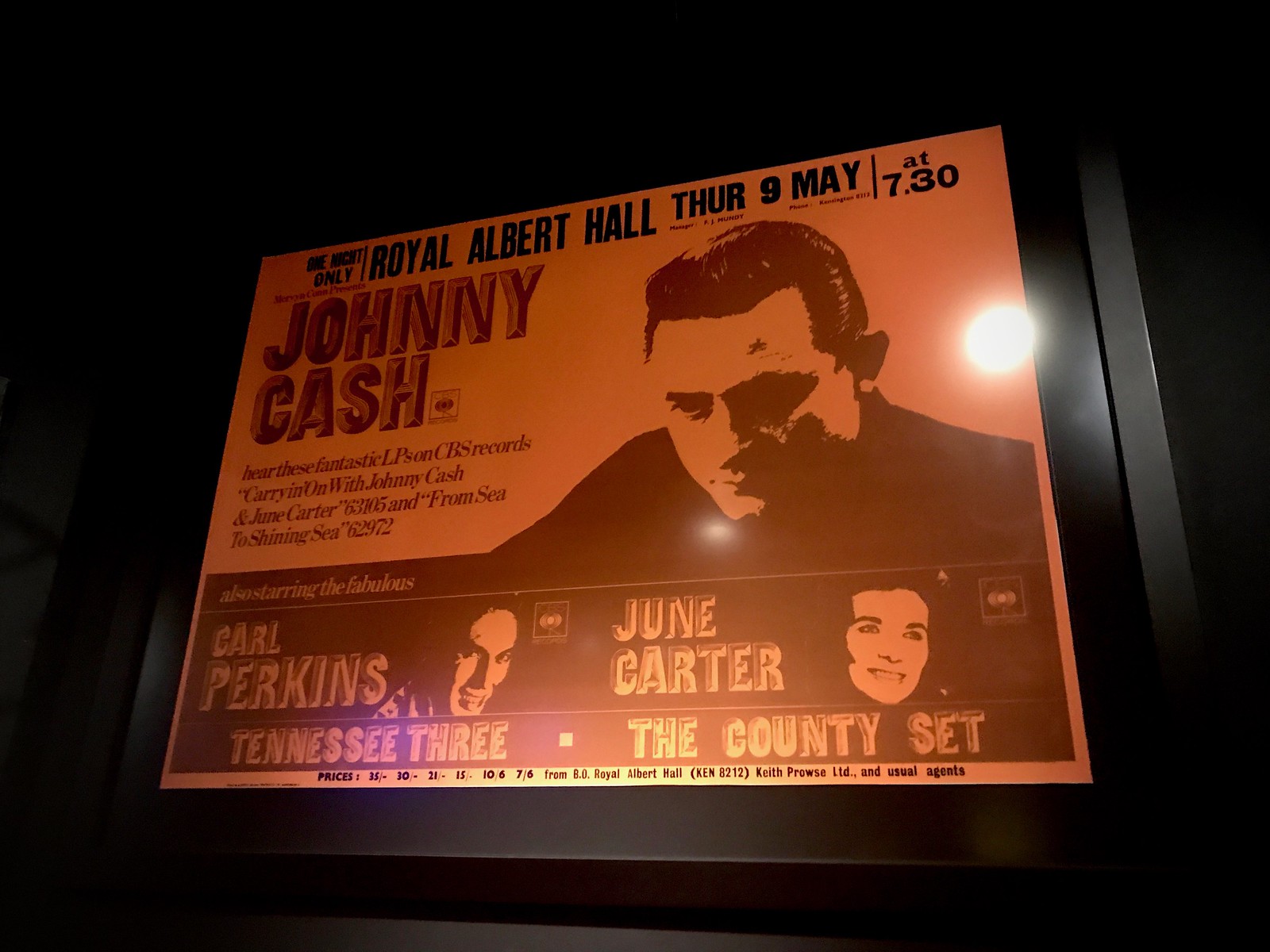The promotional flyer for the concert, displayed in a sleek black, shiny, reflective picture frame with a glossy glass or acrylic covering, features an eye-catching orange center with bold black text. The top left corner of the image appears slightly smaller due to the angle of the photograph. At the top of the poster, black text announces, "One night only, Royal Albert Hall, Thursday, 9th May at 7.30." Beneath it, in a greyish font, the name "Johnny Cash" stands out prominently. An image of Johnny Cash, with highly gelled hair and wearing a black shirt, is located in the top right corner, looking towards the bottom left of the poster.

The flyer additionally advertises performances by Carl Perkins and June Carter, with mentions of "The Tennessee Three" and "The Country Set." There is a note in black text that reads, "Here are these fantastic LPs on CBS Records." The poster's dimensions are approximately six inches wide by five inches tall, and throughout the orange rectangle, various descriptive details and print sizes emphasize the notable performers and event specifics. Towards the bottom, black and red text provides ticket prices and additional purchasing information, including "35/30, 21, 15/10, 6/7" and "from BO Royal Albert Hall (Ken 8212), Keith Prowse LTD, and usual agents."